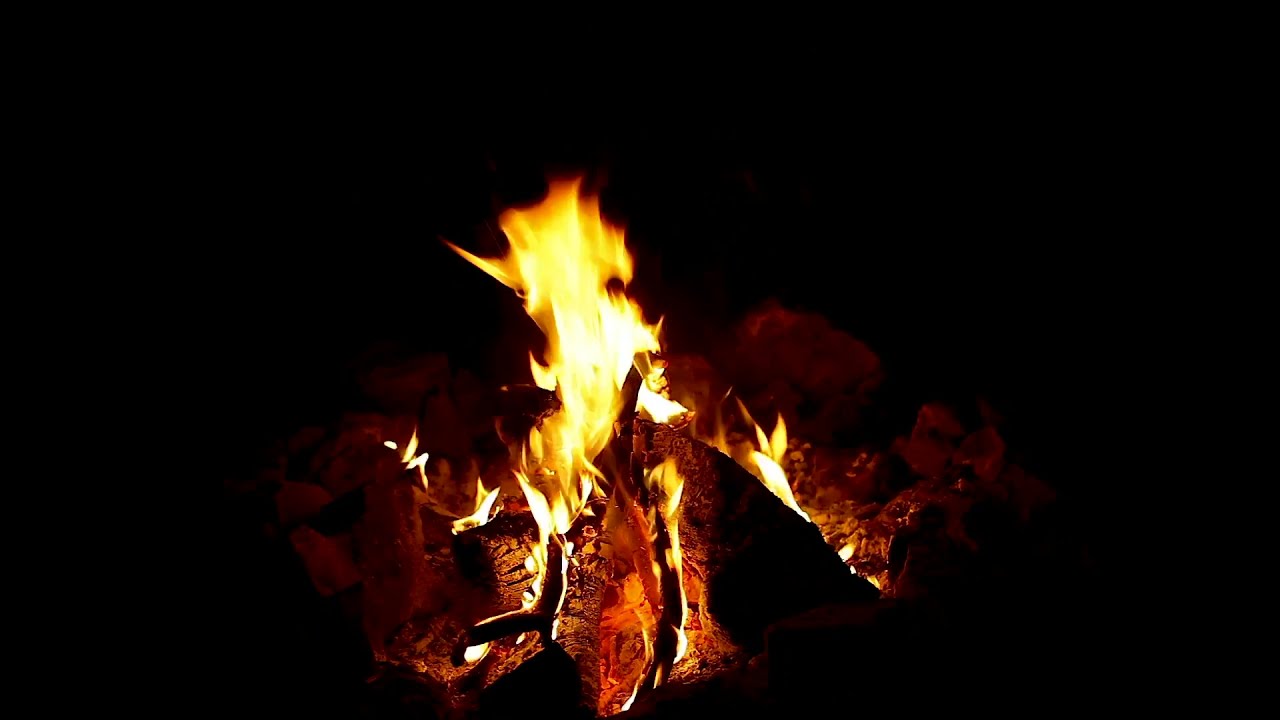The image is a striking photograph centered on a campfire, set against an all-black backdrop that emphasizes the fire's luminosity. The campfire, enclosed within a ring of stones, showcases a blend of twigs and logs that have burned down to various stages of combustion. In the core of the fire pit, thin, broken pieces of wood are alight, some covered in ash and others glowing an intense red from the heat despite having no visible flames. Towering in the center in a teepee-like formation, logs emit brilliant white and yellow flames that climb nearly three-quarters up the photograph. The scene captures the serene beauty of firelight in the dark night, with the surrounding pitch-black emptiness enhancing the stark simplicity and focused radiance of the fire itself. The overall shape of the photograph is wider than it is tall, akin to a high-definition TV screen, and it beautifully highlights the serene glow of the campfire amidst the profound darkness.